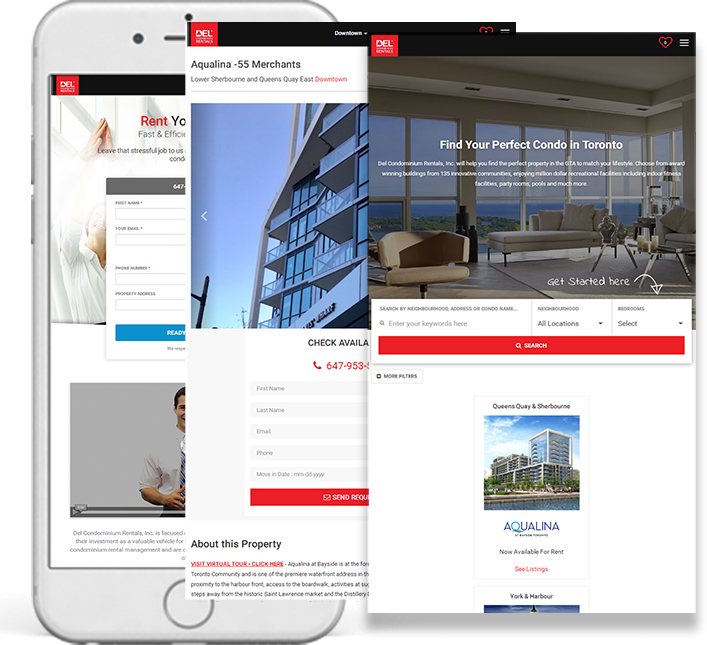This image is a collage of three overlapping screenshots from a mobile application used by real estate management companies, particularly those dealing with Toronto-based properties. The primary screenshot in the foreground features the text "Find your perfect condo in Toronto," showcasing picturesque corner-front condos that offer expansive aerial views of the cityscape, indicating high-rise living.

The second screenshot highlights a specific property, "Aqualina," located at 55 Merchants Wharf at Lower Sherbourne and Queens Quay in downtown Toronto. 

The third screenshot is focused on a contact form for rental inquiries, asking users to provide their name, email, and contact information. A smiling salesperson is also visible, reinforcing the service-oriented nature of the app. This app is designed to simplify the process of finding, renting, and managing condos in the Toronto area.